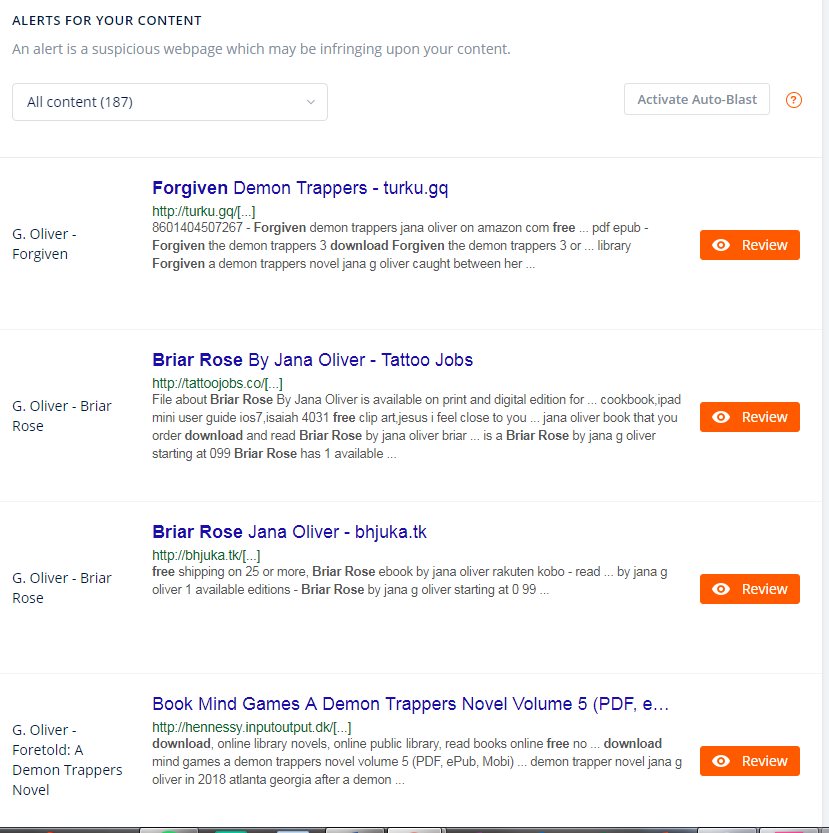This image is taken from a website that tracks potential copyright infringements, indicated by the header "Alerts for your content." This section alerts users of suspicious webpages that may be using their content without authorization.

At the top of the interface, a dropdown menu labeled "All Content (187)" allows users to filter their alerts. Next to this, a gray button labeled "Activate Auto-Blast" is followed by an orange circle with a question mark, likely offering help or additional information about this feature.

Below these controls, there's a thin gray line that segments the alert entries. Four entries are visible on the screen, each involving content attributed to "G. Oliver" but with varying details provided for each alert:

1. **G. Oliver - Forgiven (Forgiven Demon Trappers - tr.uk.gq)**: This entry provides a review option, marked by an 'i' symbol within an orange box.
2. **G. Oliver - Briar Rose (Briar Rose by Janna Oliver - Tattoo Jobs)**: Again, it offers a review option, denoted by an orange box containing the 'i' symbol.
3. **G. Oliver - Briar Rose (Briar Rose by Janna Oliver - bhjuka.tk)**: This listing also presents a review option with the same orange box and 'i' icon.
4. **G. Oliver - Foretold: A Demon Trappers Novel (Volume 5)**: The review option is similarly available with an orange box containing the 'i' symbol.

Each entry offers users the ability to review the suspicious content, allowing them to investigate potential infringements further.